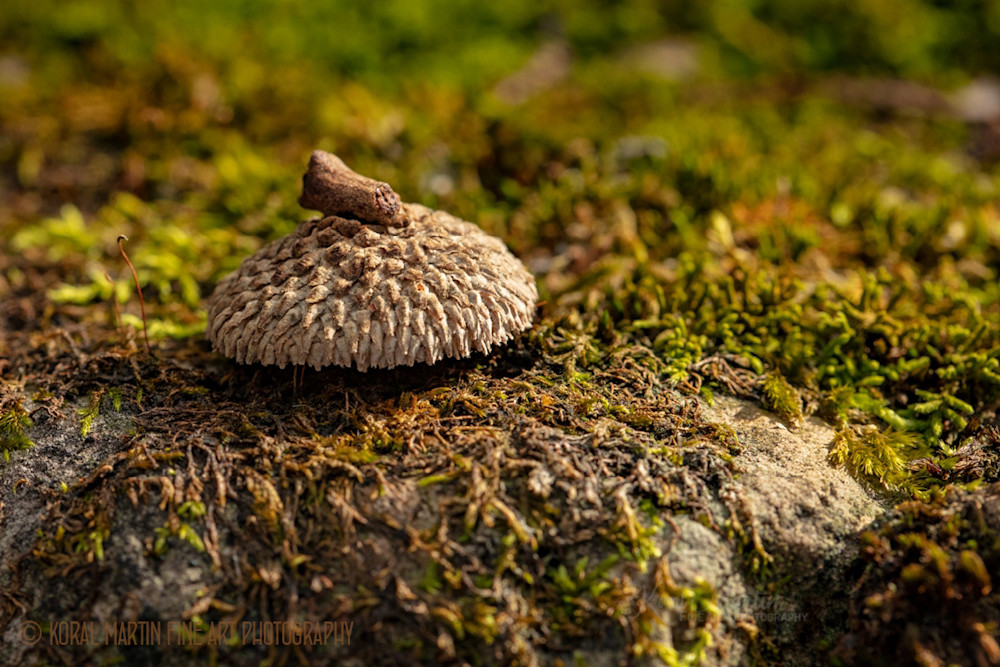The image captures an outdoor scene, focusing on the damp, moss-covered ground with a greenish-brown hue. At the center lies the cap of an acorn, a distinct light brown shade with a muffin top texture and a small stem on top, suggesting the top part of an acorn without the bottom stalk. The background, comprising green and brown vegetation resembling moss or algae, is intentionally blurred, drawing attention to the acorn cap. The ground appears muddy and moist, suggesting recent rain or high humidity. In the bottom left corner, the text "Coral Martin Fine Art Photography" in a light brown font is visible, while a barely discernible, cursive watermark in light whitish-gray occupies the bottom right corner, blending into the rock. The overall composition emphasizes the earthy, natural setting and intricate details of the acorn cap against a soft-focused backdrop.